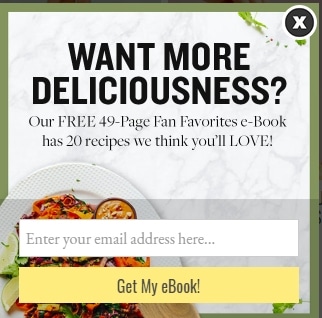The image is a screenshot of a pop-up advertisement designed to capture email addresses for a promotional offer. The ad features an olive green border with a black circle and a white 'X' in the corner, allowing users to close the pop-up. Centered against a clean white background, the headline in bold black font reads, "Want More Deliciousness?"

Below the headline, a subheader in smaller black text states: "Our free 349-page fan-favorites eBook has 20 recipes we think you'll love." The ad prominently displays an image of a plated dish featuring a variety of vibrant colors—shades of yellow, red, green, brown, and tan—served on a white plate with a subtle gray checkered pattern.

Beneath the image, there is a white text field with gray text that prompts users to "enter your email address here." Adjacent to this field, a long yellow button with gray text encourages visitors to "Get My eBook."

The overall design is simple yet effective, making use of large, easy-to-read fonts. The image also includes small green garnishes, likely parsley, enhancing the visual appeal. The pop-up is free from any other distracting elements, focusing the user's attention on the key message and call to action.